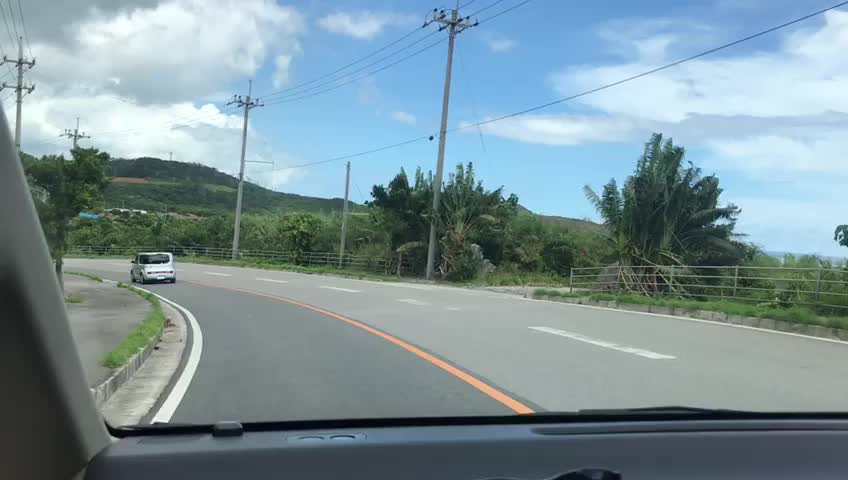This photograph, captured in landscape mode from inside a vehicle on the left side of the road, showcases a three-lane roadway that curves to the left. The image prominently features the vehicle's black dashboard at the bottom, giving a clear view through the windshield to the scenic landscape beyond. The sky, filling the top half of the image, transitions from dark gray with white clouds on the left to a bright blue with patches of white and gray clouds towards the center and right.

On the right side of the roadway, green hills blanketed in grass rise and fall, dotted with a mix of trees, including tall palm trees. These hills extend across the background, providing a lush, green contrast to the asphalt. The road surface is defined by a solid yellow line on the left edge and dashed white lines separating the lanes. The lane closest to the curb is bordered by a solid white line.

Additionally, another vehicle, likely white or silver, is visible in the same lane as the car from which the photo is taken, further emphasizing the left-side driving orientation. The combined elements of the roadway, the greenery, and the dynamic sky create a vivid, detailed scene of a drive through a picturesque landscape.